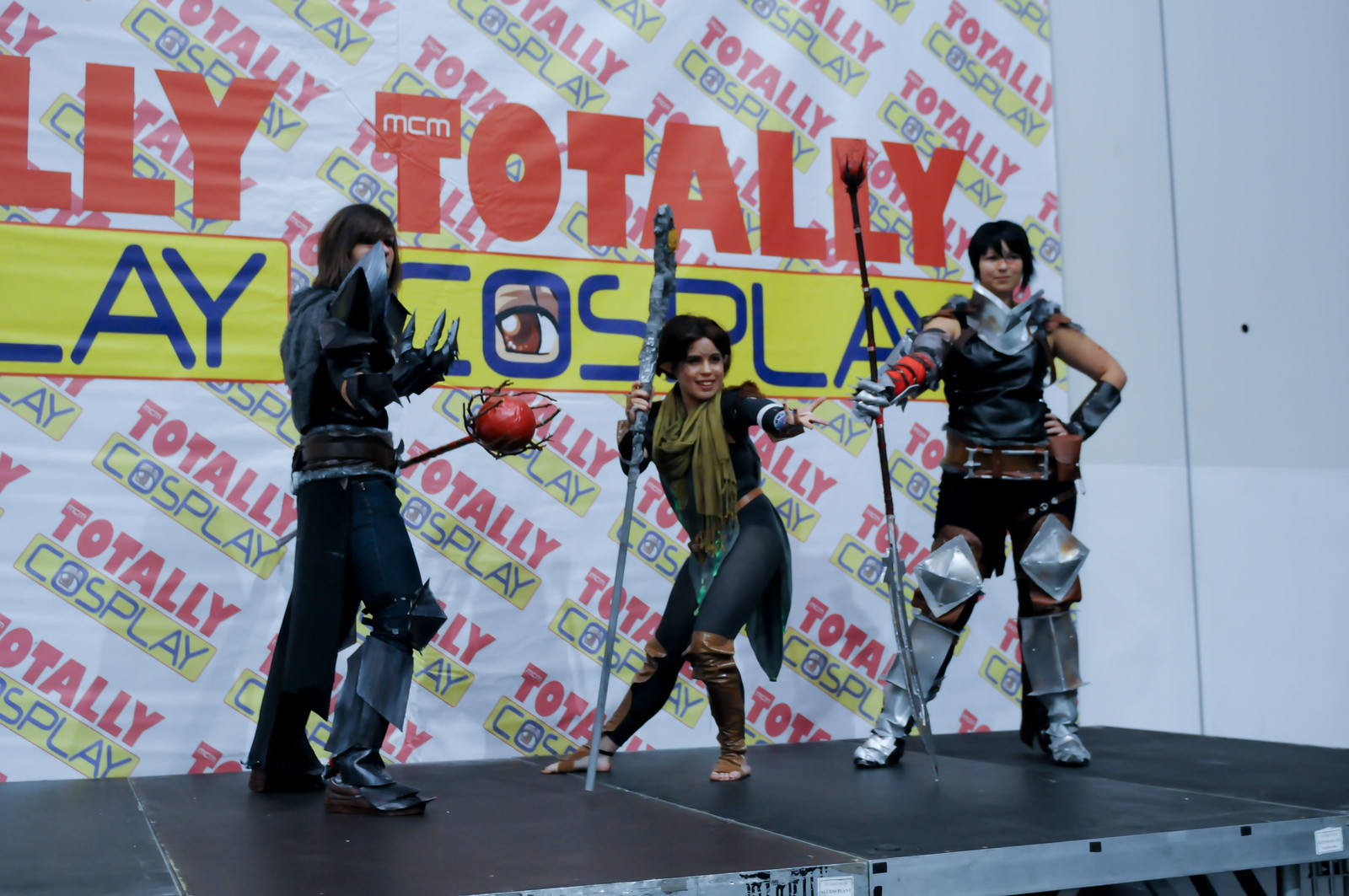This image showcases three individuals on a stage intricately designed to resemble a giant board game or video game scene. They are dressed in detailed, fantasy-inspired cosplay costumes. From left to right:

- **Person on the left:** This individual, possibly a woman, has a masked face shrouded by long hair. The gray mask complements her unique outfit, which includes a peculiar uniform with protective gear wrapped around the waist and metal-like claws on a black glove. She wields a long spear with a distinctive red ball surrounded by spikes.

- **Person in the middle:** A woman stands confidently, donning a black jersey paired with a brown scarf around her neck. She has brown and black boots and is holding a weapon that extends from the floor to several feet above her head. Her left hand is outstretched towards the front of the stage, emphasizing her striking presence.

- **Person on the right:** Another female character, outfitted in intricate gear. She wears a combination of a gray chest armor piece, a black vest, black pants, and metal shoes. Her black hair is short, and her arms are gloved differently; a blue and red striped glove on the right and a black leather glove on the left. She holds a spear featuring a double-tip design.

The backdrop is a prominent white banner with bold red and green lettering that spells out "Totally Cosplay," reinforcing the event's theme. The letters of "Cosplay" are particularly large, standing out on a yellow background. This scene epitomizes the enthusiasm and creativity of participants at a cosplay event, with attention to detail that brings their characters to life.